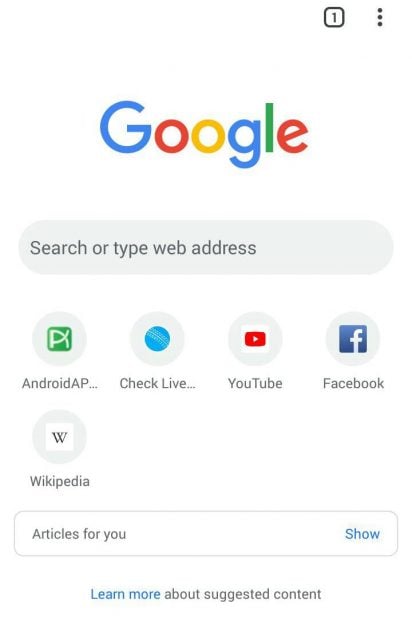This is a screenshot of a Google homepage displayed on a cell phone browser. At the very top, the browser's user interface is visible; the tab button indicates that only one tab is open. To the right of the tab button is the three-dot drop-down menu. 

Prominently, at the center top of the page, is the colorful Google logo, featuring the letters "G," "o," "o," "g," "l," and "e" in blue, red, yellow, blue, green, and red respectively. Just below the logo is the search box with a placeholder text that reads "Search or type web address."

Further down, there are shortcuts to frequently used apps or websites. The first shortcut is represented by a green thumbnail labeled "Android AP...". Next to it is a blue circle icon labeled "Check live...". The third shortcut is the YouTube thumbnail, which has the YouTube logo and the text "YouTube" underneath it. The fourth shortcut displays the Facebook logo with the text "Facebook" directly below. Lastly, on the second row to the left, is the Wikipedia shortcut featuring the Wikipedia logo and the name "Wikipedia" beneath it.

Near the bottom of the screen, there's a square box labeled "Articles for you," with a "Show" button beside it. The very bottom of the page contains a link that reads "Learn more about suggested content."